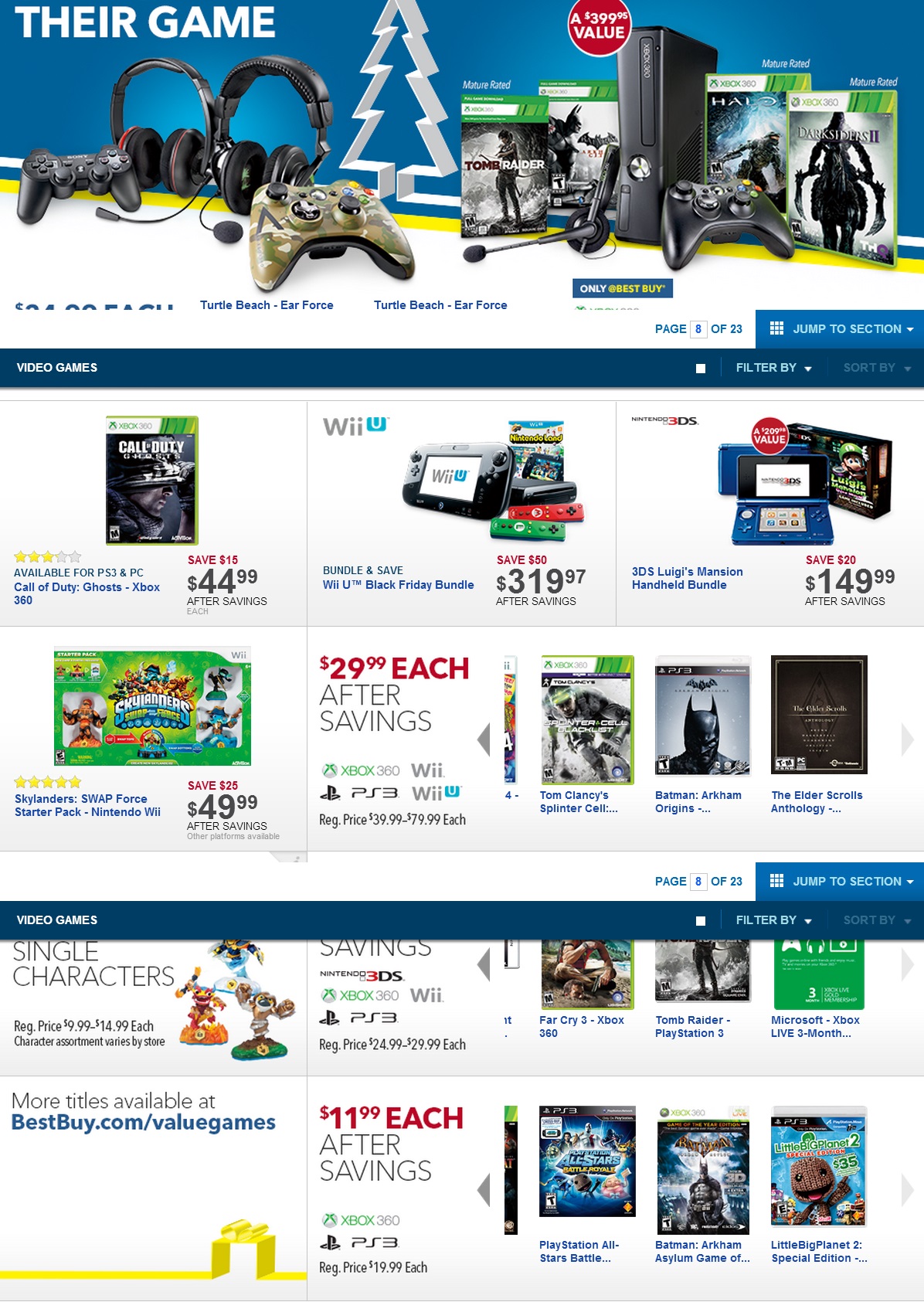Here's the cleaned-up and detailed caption:

---

This webpage from an online retailer, which specializes in gaming systems and games, features a prominently dark blue header adorned with a white Christmas tree and a cutout in the center, indicating a Christmas or pre-Christmas sale. 

On the left side of the page, there is an image showcasing various gaming accessories including two black headsets, one of which has a red accent. Adjacent to these, there is a black PS3 controller on the left and a camouflage Xbox 360 controller with a silver d-pad and black analog sticks on the right.

The right side of the page highlights a black Xbox 360 console surrounded by several game titles and a black controller. To the left of the console, there is a black headset. Above this setup, a red circle contains white text reading, "A $399.95 value," and below, it mentions "Only at Best Buy" in a dark blue rectangle. The word "Only" is in white text, whereas "Best Buy" is in yellow.

Flanking the Xbox 360 are game titles such as "Tomb Raider," "Batman," "Halo," and "Darkstalkers." Below this section, there are individual promotions: "Call of Duty: Ghost" priced at $44.99, touting a $15 saving in red text; a Wii U bundle, claimed to save $50, priced at $319.97; and a "3DS Luigi's Mansion Handheld Bundle" priced at $149.99 with a $28 saving.

Next, "Skylanders" is listed at $49.99 with a $25 saving indicated in red. The next panel mentions "$29.99 each after savings" in red text, with specific systems like Xbox, Wii, PS3, and Wii U having regular prices ranging from $39.99 to $79.99 each. 

Visuals for Tom Clancy’s "Splinter Cell," "Batman: Arkham Origins," and "The Elder Scrolls Anthology" are featured. Another section lists individual characters priced regularly between $9.99 and $14.99 each, with additional titles available at BestBuy.com/valuegames.

Additionally, there are various games listed, including "Far Cry 3" for Xbox 360, "Tomb Raider" for PS3, and a 3-month Xbox Live subscription. Savings are marked for Nintendo 3DS, Xbox 360, Wii, and PS3 games, with regular prices ranging from $24.99 to $29.99 each. The subsequent section offers games at $11.99 each after savings, with regular prices at $19.99 each, mentioning titles like "PlayStation All-Stars Battle," "Batman: Arkham Asylum Game of the Year Edition," and "Little Big Planet 2 Special Edition."